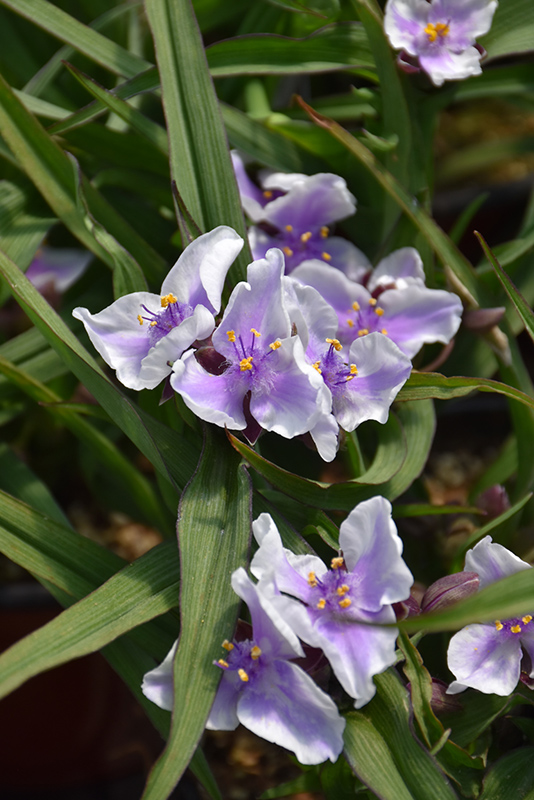The photograph is a vivid, close-up image of a vertical rectangle orientation showcasing nine stunning purple iris blooms. These delicate flowers feature richly-colored purple interiors and lighter, almost white edges on their petals, with vibrant yellow stamens at their centers, poised for pollination by bees and birds. The background is a lush mix of greenery, accentuating the irises that are scattered throughout the image. Some of the leaves exhibit a dark to pale green hue with occasional brown tinges on the edges. Additionally, small bits of debris are visible beneath the green stems, adding a natural, earthy detail to this beautiful outdoor scene.